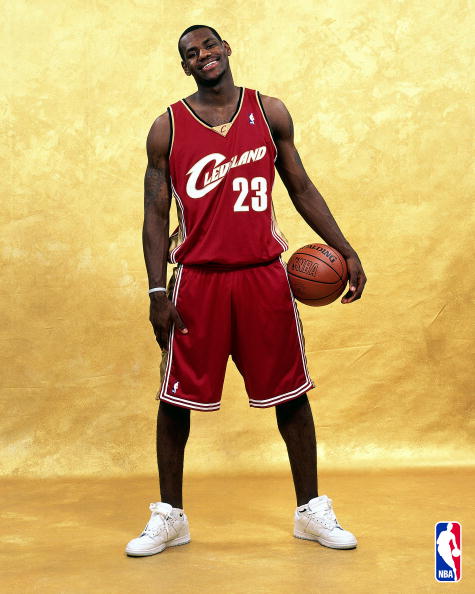The image captures LeBron James during his rookie days, posing like for a baseball card. He’s wearing a red Cleveland Cavaliers jersey with the number 23 in white lettering on the front. His matching red shorts feature white stripes along the sides. LeBron’s muscular arms stand out, and he holds an orange basketball against his left hip with his left hand, his right arm resting down by his side adorned with a white bracelet. He is smiling with his head tilted slightly to the left. He is outfitted in white Nike basketball shoes and white socks. The backdrop is a golden yellow, extending seamlessly from the floor to the wall, giving the photo a studio effect. In the bottom right corner, the iconic red, white, and blue NBA logo is visible.